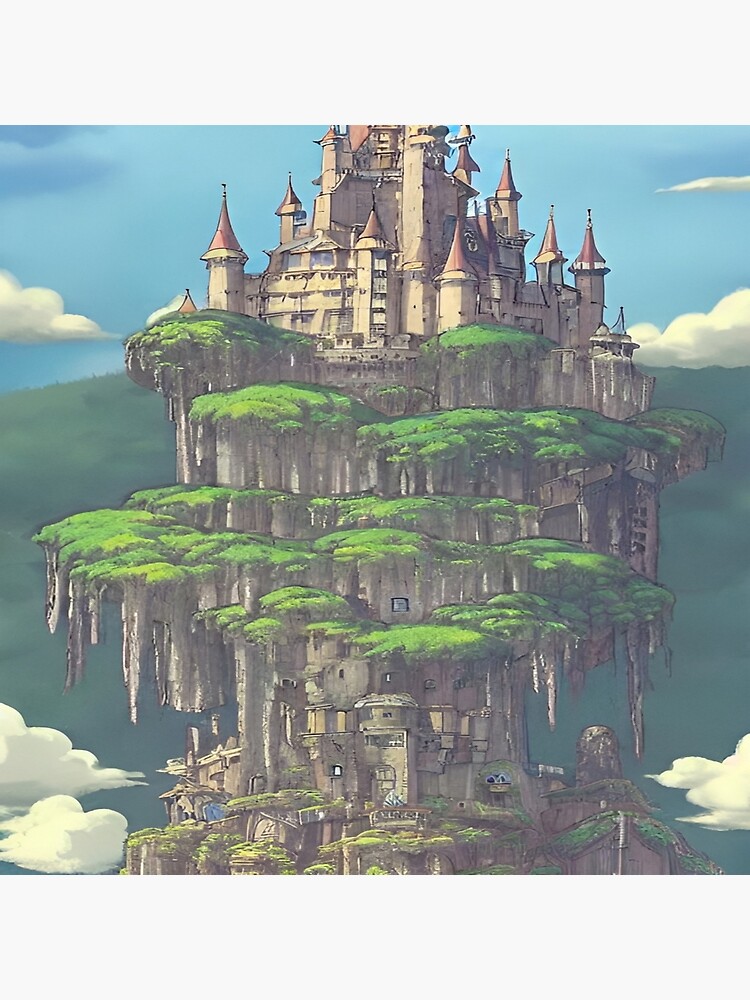This image, evocative of Studio Ghibli's whimsical and fantasy aesthetics, depicts a surreal landscape featuring a grand castle perched atop a massive, solitary mountain or tree-like structure suspended in the sky, enveloped by scattered clouds. The castle, notable for its red, pointed turrets, commands the scene from the peak, imparting a mystical aura. Below the castle, the structure descends into a cityscape that seamlessly blends into the earth-toned, moss-covered trunk or base, giving an impression of a colossal tree. The greenery clings to the edifice, resembling mossy patches, stalagmites, and rocky outcrops, suggesting a place carved painstakingly from nature itself. The background is equally enchanting, with a bright blue sky dotted with a few scattered clouds and a green, grassy hill, indicating a sunny day. Although grey and somewhat somber at parts, the vibrant greenery adds life and contrast. The entire image, painted rather than photographed, radiates the charm of a handmade illustration, capturing the essence of a fantastical "castle in the sky."